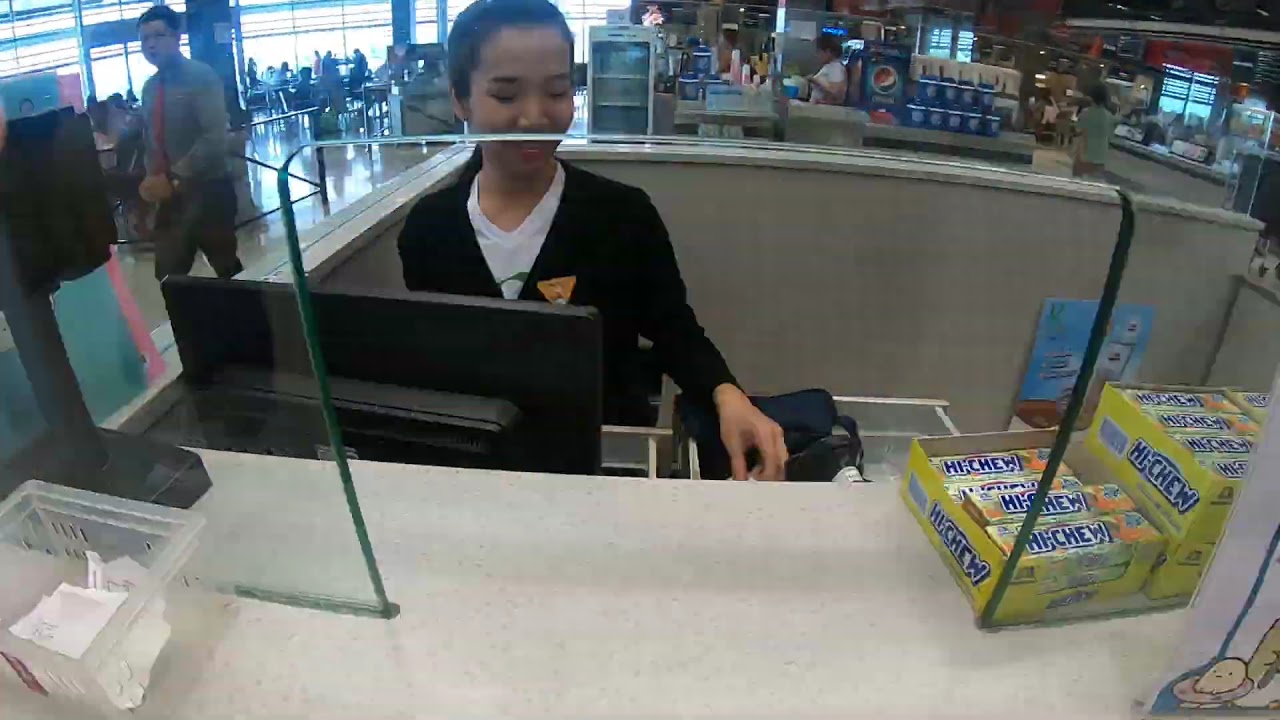In a horizontally aligned rectangular image, a woman, likely Asian with black hair pulled back, stands behind a glass window with a central opening, working at what appears to be a cash register. She is at the center of the image, dressed in a long-sleeved black jacket or cardigan over a white v-neck graphic t-shirt. With her left hand, she is accessing an open drawer in front of her, where a black computer monitor is partially visible from the back. To the right of the frame, various boxes of Haichu candy are neatly arranged. On the left, an acrylic white box holds various pieces of scrap paper. 

Behind her, the backdrop reveals a bustling food court area with people sitting at benches and tables, engaging in different activities. In the top left corner, a man wearing a long-sleeved gray dress shirt with a tie and black slacks can be seen walking. Also visible are Pepsi-Cola cans and a large wall of windows bathed in light, enhancing the lively ambiance of the scene.